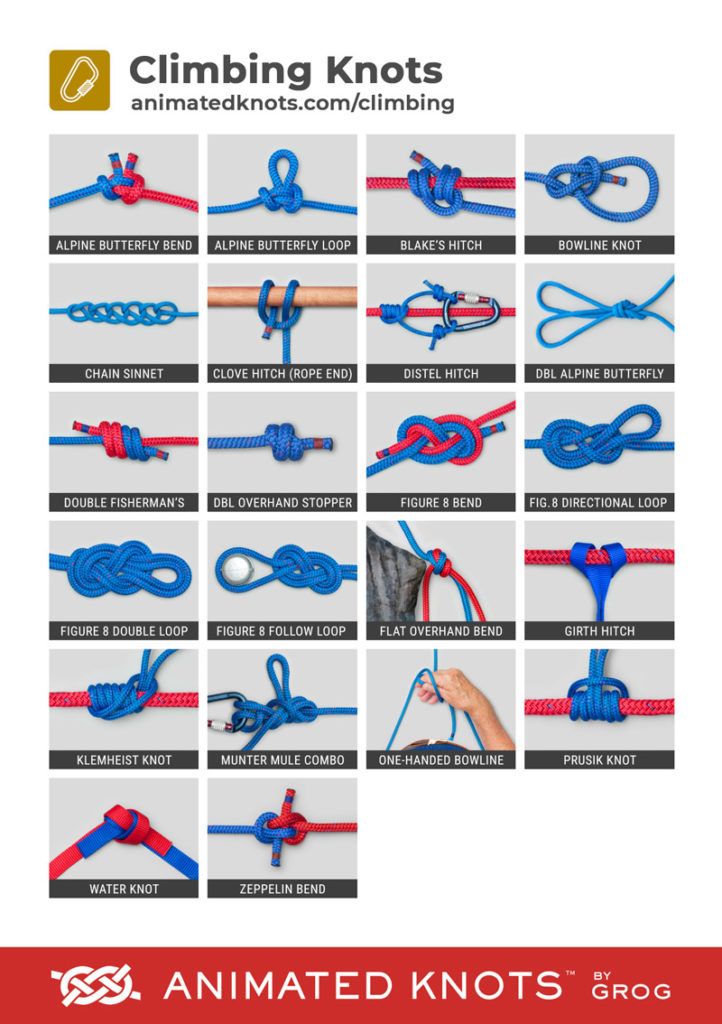This is a comprehensive infographic poster on Climbing Knots, presented on a white background. At the top, there is a gold square featuring a carabiner, accompanied by the title "Climbing Knots," followed by the URL "animatedknots.com/climbing" in black text. The main section displays a series of knots arranged in a grid format, with each square showing a different knot tied with red or blue string, set against a light gray background. Each knot is labeled below in a black rectangle with white text.

The knots featured include: Alpine Butterfly Bend, Alpine Butterfly Loop, Blake's Hitch, Bowline Knot, Chain Sinnet, Clove Hitch, Distel Hitch, Alpine Butterfly Knot, Double Fisherman's, Double Overhand Stopper, Figure 8 Bend, Figure 8 Directional Loop, Figure 8 Double Loop, Figure 8 Follow Loop, Flat Overhand Bend, Girth Hitch, Kleimheist Knot, Munter Mule Combo, One-Handed Bowline, Prusik Knot, Water Knot, and Zeppelin Bend. Notably, some knots incorporate additional tools such as a carabiner, a wooden dowel, or a hand for demonstration.

At the bottom of the poster, a red horizontal rectangle features a white cartoon knot with the text "Animated Knots by Grog."